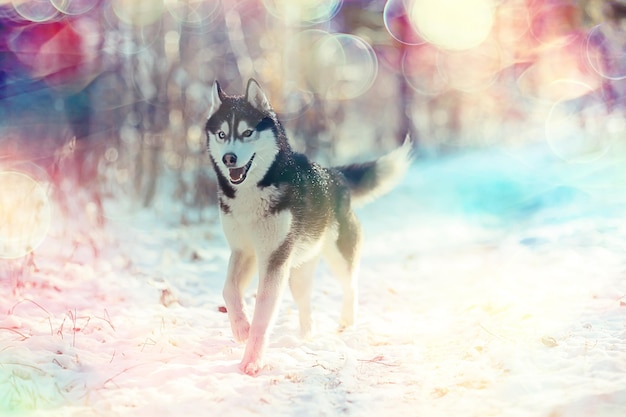This close-up photograph captures a striking image of a Siberian Husky, possibly an Alaskan Malamute, standing outdoors in a snowy landscape. The dog, with its distinctive black and white fur, is centrally focused in the image, appearing as if about to start running, facing slightly toward the bottom left corner. The Husky's eyes are heterochromatic, with one dark blue and the other seemingly white. The intricate details of the fur show a stark contrast between the dark black on the top of the body and around the head, and the clean white under the body, legs, and tail tip. The dog's expressive face is adorned with a blackish pink nose, white furred ears, and a visible, joyful expression with what looks like a big smile.

The setting is a lightly snow-covered ground with a few blades of grass poking through and blurry tree trunks in the background, indicating a wooded area. The entire background of the photograph is out of focus, accentuating the central figure of the Husky, with blurred colorful lights resembling bokeh effects scattered across it. A filter has been applied, creating a rainbow-colored haze and lens flares primarily around the top corners, adding a dreamy, ethereal quality to the snowy scene. Sunlight filtering through the trees enhances the magical atmosphere of the image.